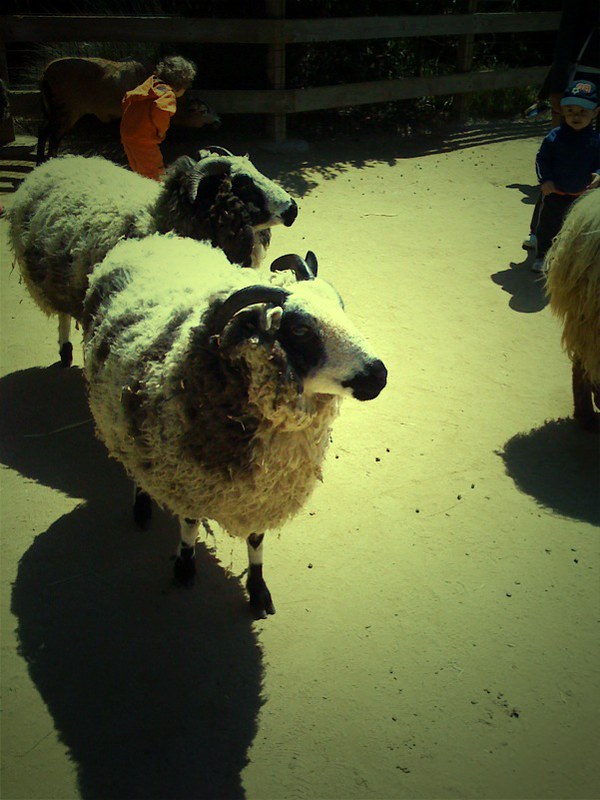This photograph, with a muted and slightly yellow-tinged color palette, captures a lively scene at what appears to be a farm or nature reserve. The primary focus is on two woolly rams positioned slightly to the left of center. The foremost ram is mainly white with distinctive black patches, including a patch over its eye, a black nose, a patch on its shoulder, and black markings around its feet and ankles. Behind it, another ram, partially obscured, appears somewhat greyer due to the lighting, but shares a similar white woolly coat and sports dark horns.

In the background, among the sand and casting dramatic shadows, are people and children, adding to the bustling atmosphere of the setting. To the top right of the frame, a small child dressed in a blue coat and cap, likely around 5 or 6 years old, is seen sitting on a tricycle. Another child, similarly aged, can be seen further back, donning an orange jacket and bending down to look at a dark animal, possibly another sheep or a cow, though the poor lighting makes it hard to distinguish.

Additional subtle details enrich the scene: the blackish shadows of the rams, the textured fur illuminated by sunlight, and various clothing colors, including the navy blue and yellow of a baseball cap and the stark orange jacket. The entire scene is framed by horizontal fencing at the back, and the once vibrant colors now muted, suggest an aged photograph.